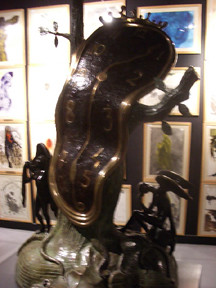This detailed photograph captures a striking scene inside what appears to be a museum or an art gallery. The image prominently features a three-dimensional, bronze or brass-colored sculpture of a ruffled-shaped spherical clock face. The clock face is black with gold trim and gold numbers clearly visible from 1 through 12 around its edge. Long, gold-colored hands adorn the face, which looks dramatically extended and melted, evoking Salvador Dali's iconic "Persistence of Memory."

On top of the clock is an ornate crown, while tree branch-like elements emerge from the sides of the clock face, with one particularly resembling an arm or limb. The lower part of the sculpture has a more grayish hue, enhancing the surreal, almost organic feel of the piece.

In the background, the dark wall is adorned with several gold-framed artworks, including paintings and drawings. The paintings predominantly feature dark colors, except for a notable blue one resembling Van Gogh's "Starry Night." These artworks are arranged in columns, adding depth to the scene as they extend vertically, and some are partially obscured by the sculpture, emphasizing its prominence.